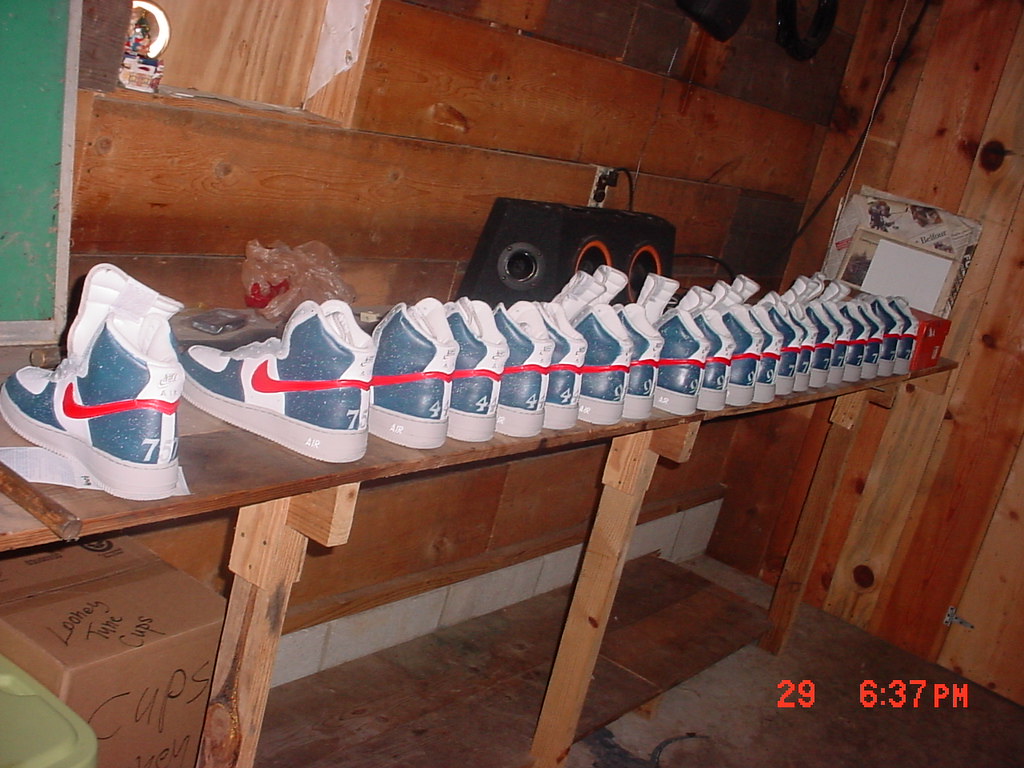This photograph captures a lineup of nearly 25 identical Nike high-top sneakers arranged meticulously on a wooden shelf, supported by sturdy homemade wooden posts. Each sneaker is predominantly dark speckled green with white accents and features a distinctive red Nike swoosh. The shoes display double-digit numbers on the back, likely indicating team uniform numbers rather than sizes. Positioned in a precise row facing away from the camera, the shoes are thoughtfully organized with numbers such as 00, 04, 07, and 09 recurring. The background reveals a wooden wall, suggesting the setting might be an old shed or a rustic room. To the lower left of the frame, a cardboard box with "Looney Tunes cups" can be seen, while the lower right shows a digital display reading 6:37 PM. Additional elements in the scene include speakers and a sealed window adorned with a small snow globe, adding a quaint touch to the overall ambiance. The lighting appears artificial, providing a somewhat dim and intimate feel to the image.